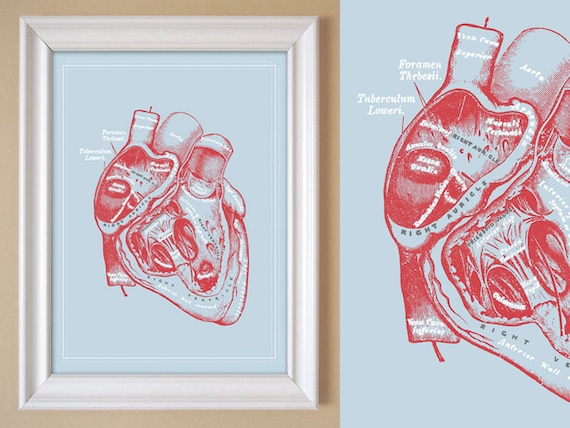The image depicts a framed, hand-drawn anatomical heart set against a blue background. The frame itself is white and hangs on a tan wall. The heart, drawn in red ink or marker and highlighted with white, is illustrated with precision, resembling a diagram one might find in a science textbook. On the left side, the entire framed picture is visible, while the right side features a close-up of the heart, making it easier to read the labels pointing to different parts of the heart. Despite the small font, the labels in white font include terms like "aorta," indicating the anatomical focus of the drawing. Overall, the image provides a detailed representation of the heart's structure, enhancing its educational value.